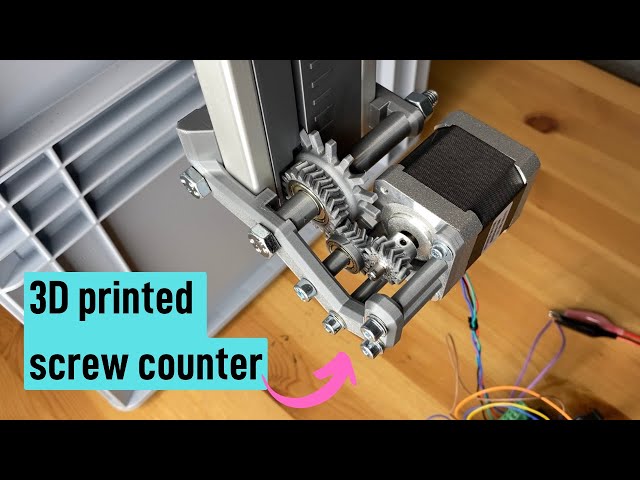This photograph features a 3D printer with a prominent focus on a 3D printed screw counter, as indicated by the label "3D printed screw counter" in the bottom right corner, highlighted by a pink arrow pointing toward the apparatus. The machine rests on a wooden floor, partially depicted in the image. Centered in the frame, various machinery components are visible, including several gears and an arm that slides vertically, adorned with large bolts. The 3D printer itself is partially out of the shot, but its base appears gray with several colorful wires—orange, yellow, turquoise, purple, pink, and more—emanating from the front, cascading onto the wooden floor. To the left side of the photo, part of a shelf is visible.